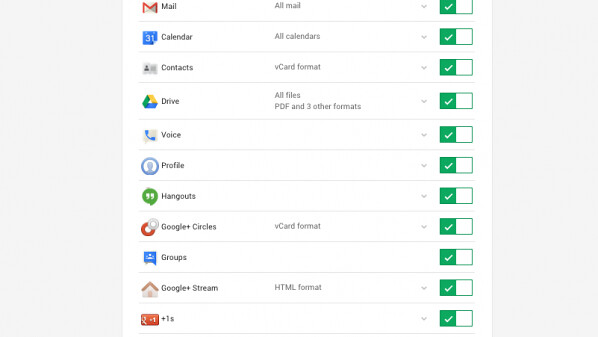This image depicts a computer screen displaying a user interface predominantly in a light gray color. In the center, there is a white square table organized in a grid format. The table comprises a list of Google products, each with an associated icon on the left. The listed items include "Mail," "Calendar," "Contacts," "Voice," "Profile," "Hangouts," "Google Plus Circles," "Groups," "Google Plus Stream," and "Plus 1S."

On the right side of each product name, there is a secondary column with further details: "Mail" has "All Mail," "Calendar" has "All Calendars," "Contacts" specifies "vCard Format," and "Drive" indicates "All Files, PDF, and three other formats."

Additionally, there are clickable indicators along the row—green checkboxes on the left and possibly changeable icons (from green checkboxes to red Xs) on the right—implying status toggles or selection options for each product. The organized layout and recognizable Google product icons suggest this is part of a Google suite interface, likely involving settings or permissions for the various services listed.